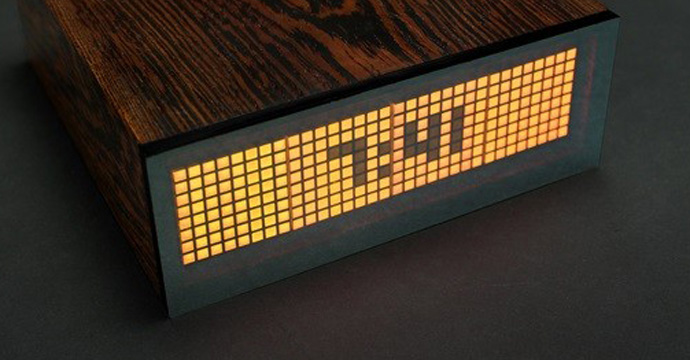This image features a contemporary digital clock with a sleek, modern design. The clock is primarily composed of a black rectangular frame and contains another black rectangle within it. The inner rectangle is artistically patterned with squares in various shades of gold and tan, creating a visually appealing mosaic effect. At the center, the time "7:41" is prominently displayed, with the digits formed from brown squares that contrast distinctly against the gold squares, ensuring readability. Notably, there is no indication of whether the time is a.m. or p.m. The clock is supported by what appears to be a wooden block and is set against a black, solid surface, possibly a table or countertop, providing a sturdy and stylish backdrop.